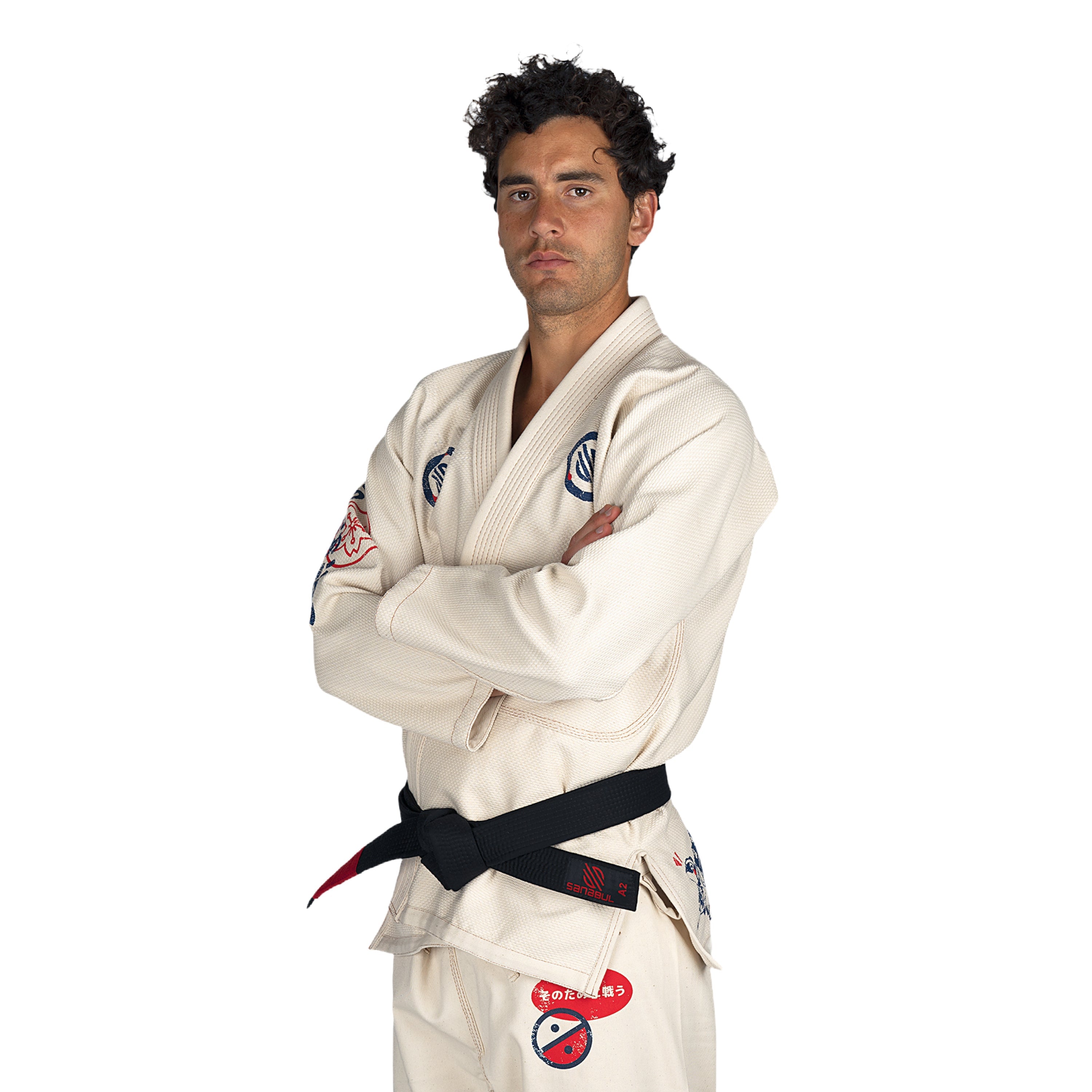This is a detailed photograph of a young man with slightly wavy black hair and a light mustache, dressed in a traditional martial arts uniform. He stands with a serious expression, his dark eyebrows and eyes conveying confidence, while his body is angled slightly to the left. His arms are crossed firmly across his chest, partially obscuring his white collarless top, which resembles a robe, typical of judo or karate. 

The uniform is adorned with various emblems. On either side of his chest are blue and white badges, while his right arm features another emblem incorporating red. His black belt, tied securely at the front, displays small red logos at the ends. His white pants are marked with distinctive patches: a red oval containing white writing on the front of his left thigh, partially hidden by his top, and a circular emblem farther down, divided into a top white half and bottom red half, with a black line and dots at the center. The circular patch is positioned at a slight angle towards the left, adding to the intricate detail of his attire. There is no background in the photograph, allowing the focus to remain entirely on the man and his martial arts uniform.